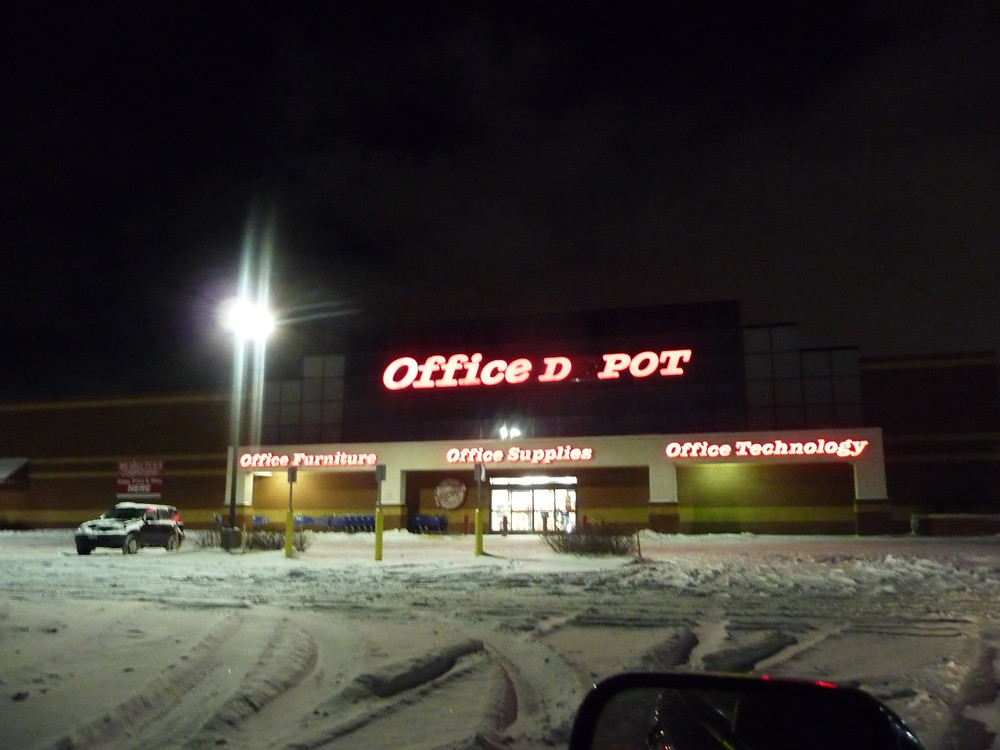This night scene captures a snowy parking lot outside an Office Depot store, taken from the passenger's window with a glimpse of the rearview mirror in the lower right corner. The parking lot, covered in snow with visible tire tracks, seems drivable, suggesting a recent plow. The Office Depot building is the focal point, illuminated against the black night sky. The main sign displays "Office Depot" in varied text styles, with the 'E' in "Depot" notably burned out, so it reads "Office D pot." Below the sign, three sections are identified by brightly lit white labels: Office Furniture, Office Supplies, and Office Technology, with LED lights enhancing visibility. The scene is complemented by a large light mount on the left, shedding light on the snow-covered cars and the store, embodying winter's grip on a bustling commercial spot.